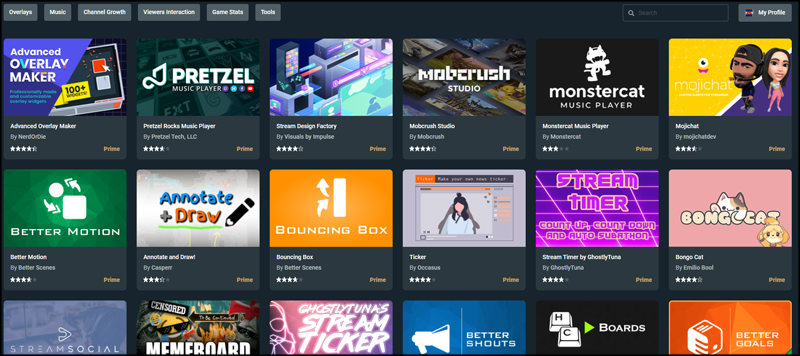Screenshot of a desktop application interface with a dark blue-black background. The interface hosts various features such as options for overlays, music, channel growth, viewer interaction, game slides, and tools. Prominently displayed are the "Search" bar and "My Profile" bar at the top. Below these, several application icons are shown in a grid format. Each box contains the app's name, an accompanying icon image, and a rating. The word "Prime" is highlighted in orange text within each app box, contrasting with the white ink used for the other text elements. Featured applications include:

- **Advanced Overlay Maker**: An app for creating advanced overlays for streams.
- **Pretzel Music Player**: A music player designed for streamers.
- **Stream Design Factory**: An app for designing stream layouts.
- **Moby Crash Studio**: A studio tool for streaming enhancements.
- **Monster Cat Music Player**: Another music player optimized for streaming.
- **Better Motion**: Possibly an app for motion graphics.
- **Annotate and Draw**: An app for annotation and drawing during streams.
- **Bouncing Box**: An interactive streaming tool.
- **Seeker**: Likely a search or discovery tool within the app ecosystem.
- **Streamer Timer**: A timer tool for streamers.

Each app appears to cater to enhancing the streaming experience through various functionalities like music integration, graphic design, interactive tools, and viewer engagement.